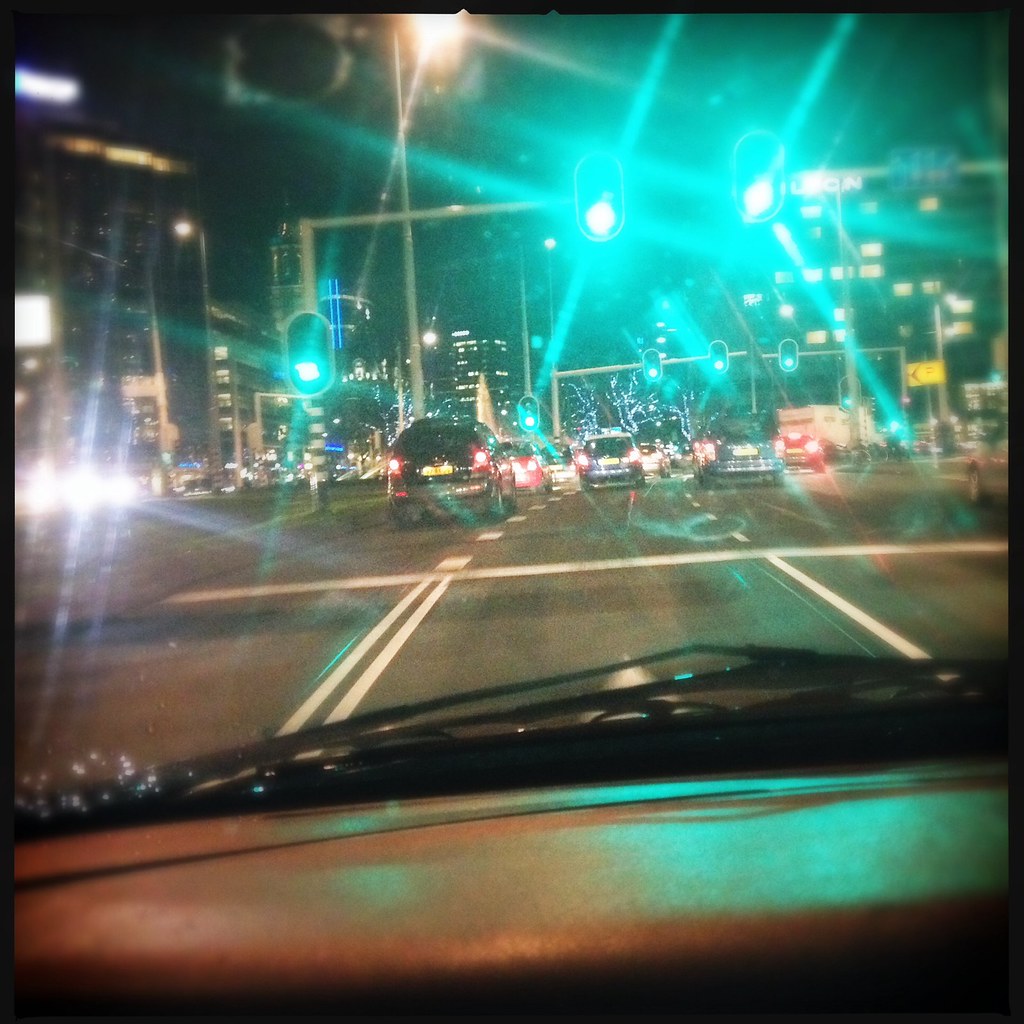A nighttime photograph taken from inside a car captures an urban intersection through the front windshield, distinguished by a brown leather dashboard partially visible at the bottom of the image. The dashboard, windshield wipers, and part of the vehicle's hood frame the view of a bustling city street. The green traffic lights dominate the scene, casting a noticeable green hue and creating pronounced lens flares that scatter across the photo. This busy three to four lane road is filled with various vehicles, including a black SUV and a red sedan with their brake lights on. Oncoming traffic from the left adds to the lens flare effect with glaring headlights. The cityscape is further defined by large buildings in the background, where some office windows are illuminated, contributing to the nocturnal city ambiance.